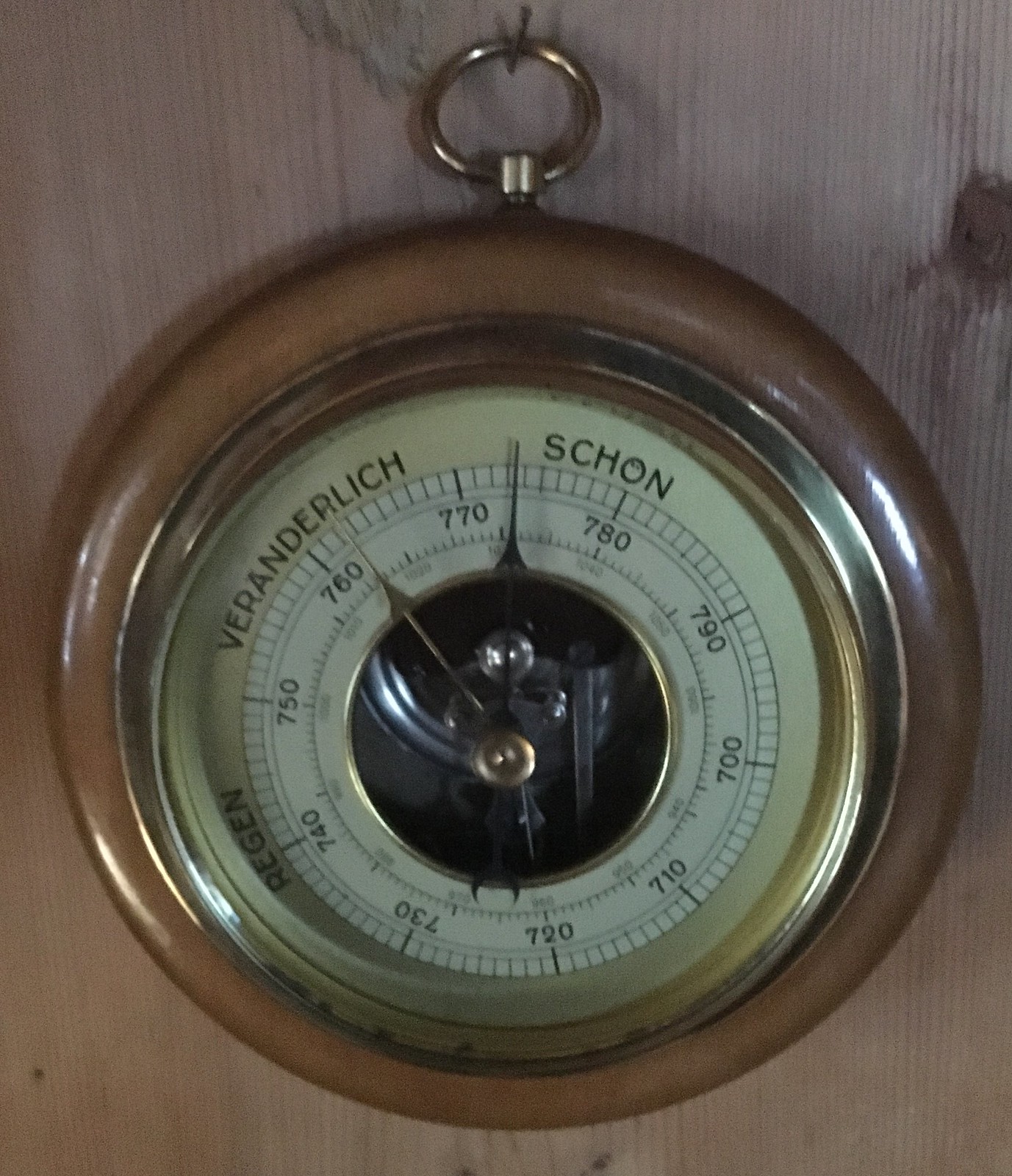Hanging on a rustic, unfinished wooden wall with pronounced wood grain, there's an intriguing, round object mounted on a single nail. The object resembles a pocket watch at first glance but is larger and not a timepiece. It features a golden brass hook connecting it to the nail. The main body of the object is metallic with a light brown hue, while the central portion showcases a lighter beige face adorned with intricate markings.

Around the perimeter, the face is inscribed with what appear to be German words, "Veränderlich" and "Schone," along with "Region." The object includes a series of numbers ranging from 700 to 790, interspersed with smaller markings. Delicate hands or pointers extend from the center, suggesting the object measures or indicates something, possibly related to climate or atmospheric conditions. Additional gears or mechanical elements are visible in the center, adding to its complex and enigmatic appearance.